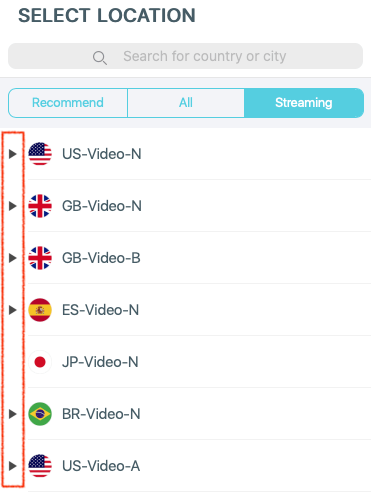At the top, in black bold capital letters, it says "SELECT LOCATION". Below this title is an elongated, light gray search bar with a magnifying glass icon on the left side. Inside the search bar, in a soft gray font, it reads "Search for country or city". 

Directly underneath the search bar, there are three clickable options, each outlined in light blue. The options are:
1. "Recommended" on the left.
2. "All" in the center.
3. "Streaming" on the right.

Below these options are a series of entries, each having a play button on the left and a flag beside it, alongside their labels:
- The first entry features an American flag with the description "US-video-in".
- The second entry shows a British flag labeled "GB-video-in".
- The third entry, again with a British flag, corresponds to "GB-video-B".
- The fourth entry has a Spanish flag labeled "ES-video-in".

Finally, at the bottom, there is an entry without a play button. Instead, it displays a white circle with a red center (the Japanese flag) and is labeled "JP-video-in".